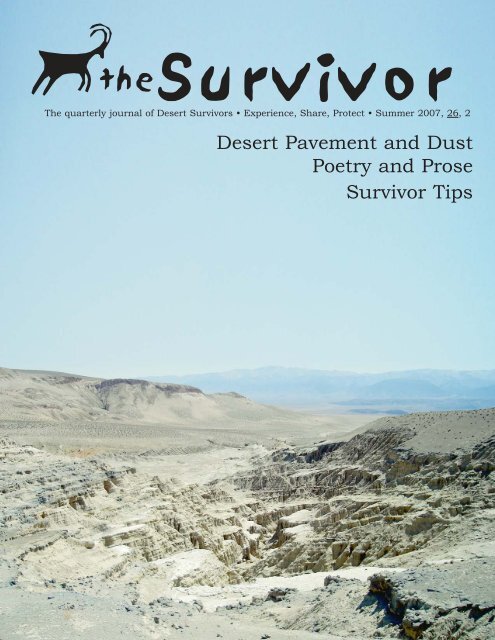This is an image depicting the cover of a magazine titled "The Survivor," a quarterly journal dedicated to desert survival enthusiasts. The cover features a photograph of a deserted canyon or mountain range, characterized by sandy or gravelly terrain with a vast, pale blue sky occupying much of the frame. Prominently displayed in black text at the top of the image are the title and subtitle: "The Survivor, The Quarterly Journal of Desert Survivors, Experience, Share, Protect, Summer 2007, 26-2." Additional text on the cover highlights the contents of the journal, including "Desert Pavement and Dust," "Poetry and Prose," and "Survivor Tips." The cover also features an image of a longhorn goat, enhancing the rugged and remote ambiance of the publication, which caters to those who engage in hiking and camping in extreme, arid environments.